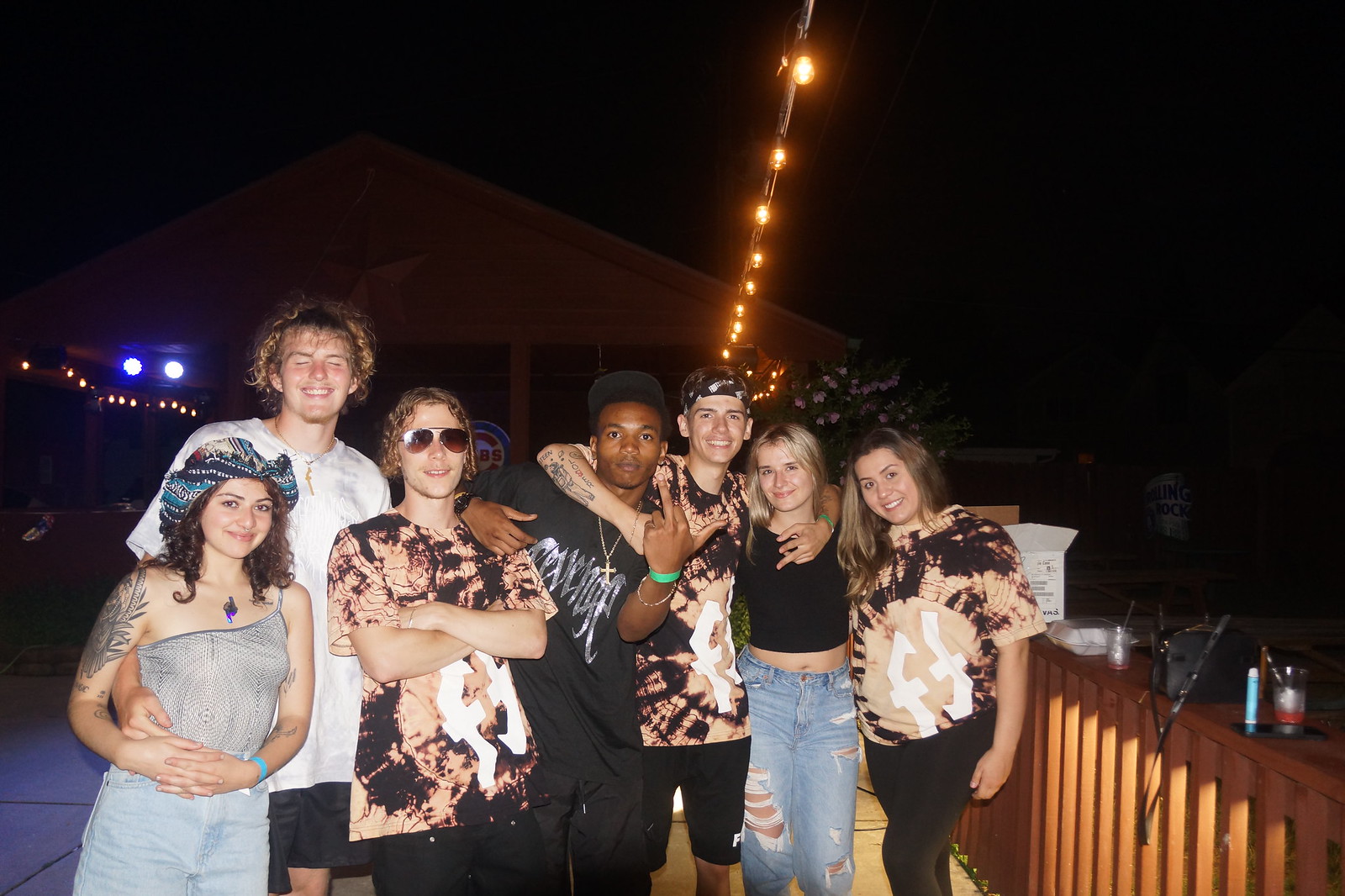This nighttime photo captures a lively group of seven young adults posing together on a wooden back porch, perhaps outside of a bar or a house. The sky is pitch black, and orange string lights hang overhead and along the edge of the building, which has an open-window design and a star emblem near the gable. The exterior appears rustic with its brown wooden structure. The group, a mix of three white girls, three white guys, and one black guy, exudes camaraderie and joy, with most of them smiling broadly.

Starting from the bottom left, a young woman is seen in denim jeans and a denim sundress, distinguished by a large flower tattoo on her right shoulder. Beside her, a taller white male with curly blonde hair is dressed in a giant white t-shirt and black shorts, affectionately holding her around the waist. Next to him, a slightly shorter young man wears sunglasses, a black and pink t-shirt, and black pants. To his right, the black male, central to the group, sports a black t-shirt, gold cross necklace, black shorts, and a green wristband, striking a playful pose with his middle finger up. Continuing right, another male also in a black and pink t-shirt and bandana smiles brightly. Adjacent to him, a girl wears a black t-shirt and blue denim jeans, stylishly cut on the sides. The final person, a long-haired woman, dons black pants and a matching black and pink t-shirt, similar to those in the group.

The friends, appearing to be in their early twenties, are dressed casually in denim, t-shirts, and shorts, radiating a warmth that contrasts with the cool night backdrop. The frequent themes of tie-dye styled shirts, bandanas, and long curly hair tie the group's aesthetic together.